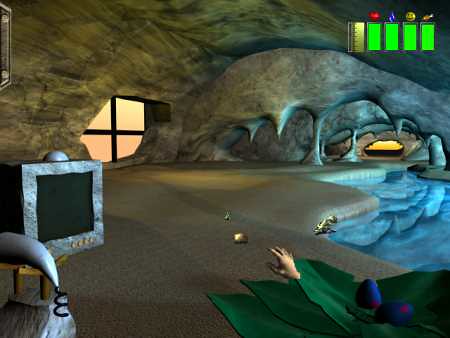The image is a horizontal rectangle resembling a scene from a vintage first-person RPG or adventure video game, noted for its roughly 20-year-old graphics characterized by blurry textures and a low polygon count. The setting is inside a gray cave with various elements establishing an immersive environment. On the left side, a window with a black cross-frame reveals a reddish-yellow sky outside. Below this window, there's a gray-outlined TV-like monitor with a black screen and four yellow buttons on the front, perched on a concrete stand with wooden legs and top. 

In the cave’s bottom left corner, near the TV, there might be a gray phone with an earpiece. Ascending from the bottom and wrapping around the scene is the cave wall adorned with stalactites hanging down from the top left. The entrance to the cave, delineated with stalagmites and stalactites, is located toward the back right.

A notable feature on the far right includes a brown object with specks of gold. Beneath it is a small body of water. Near the bottom right corner, green leaves peek out, with one gray leaf holding two blue eggs and two extending green leaves. A character’s hand, draped in a green cape, is visible in the lower right, suggesting the player's perspective.

In the top right corner, there are three power bars with associated icons: a yellow bar with a heart, a green bar with water, and another green bar possibly indicating health or another metric, accompanied by a smiley face. A chicken leg icon sits above another green bar, suggesting food or energy status. This detailed, yet pixelated, artwork convincingly transports viewers into an archaic digital cave scene punctuated by the interface elements of an older video game.